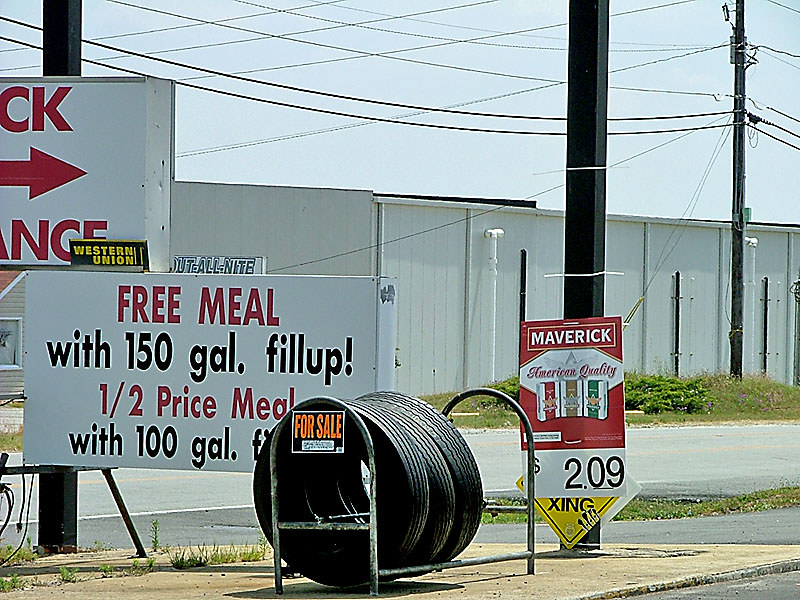In the image, tall black poles dominate the foreground, while a white building serves as the backdrop. On the left side, a partially visible sign prominently reads "Western Union" on the lower corner. Just below this, another sign offers promotional deals: "Free meal with 150 gal fill up" and "Half price meal with 100 gal," with the remaining text obscured. The words on this sign are strikingly red and black. Adjacent to these signs is a rack displaying three tires, clearly labeled "For Sale" on its front. Additionally, one of the black poles is adorned with a Maverick sign, which boasts "American Quality" cigarettes priced at $2.09 for a pack of three. The sign visually represents the three cigarette packs as well.